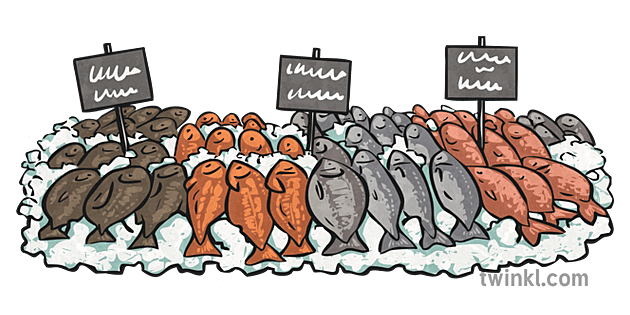The image depicts a simplistic, cartoon-like drawing of dead fish arrayed on a bed of ice, set against a white background. Each group of fish is distinctly colored and organized in rows: the far left features a row of flat-looking brown fish, followed by a grouping of more orangish-brown fish, then gray fish, and finally darker orange fish with a bit of gray in the upper right corner. Scattered across three different positions on the ice are signs with illegible white scribbles. In the bottom right corner of the image, the text "twinkle" is written without a dot com. The entire scene appears to represent a market setting, possibly illustrating the various fish types for sale.